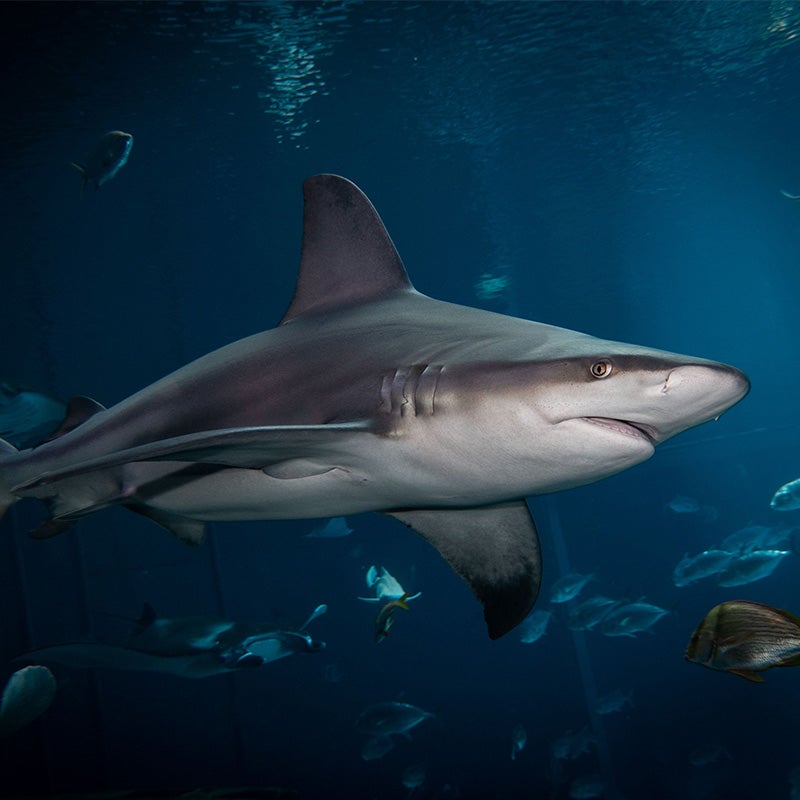In this striking underwater scene, a highly detailed image captures a great white shark swimming from left to right in profile, dominating the center foreground. The shark, illuminated against a dark, deep blue backdrop, showcases its large, iconic dorsal fin, yellowish eyes, and distinct gill slits. Its gray back contrasts sharply with its white underbelly. Surrounding the shark are various smaller fish of multiple species, adding dynamic movement to the scene. The dark waters subtly ripple and a suggestion of a reflection is seen above the shark's dorsal fin. The background fades into shadows, highlighting the shark as the focal point, with parts of its back tail cropped out. No text or additional descriptions are present in the image.